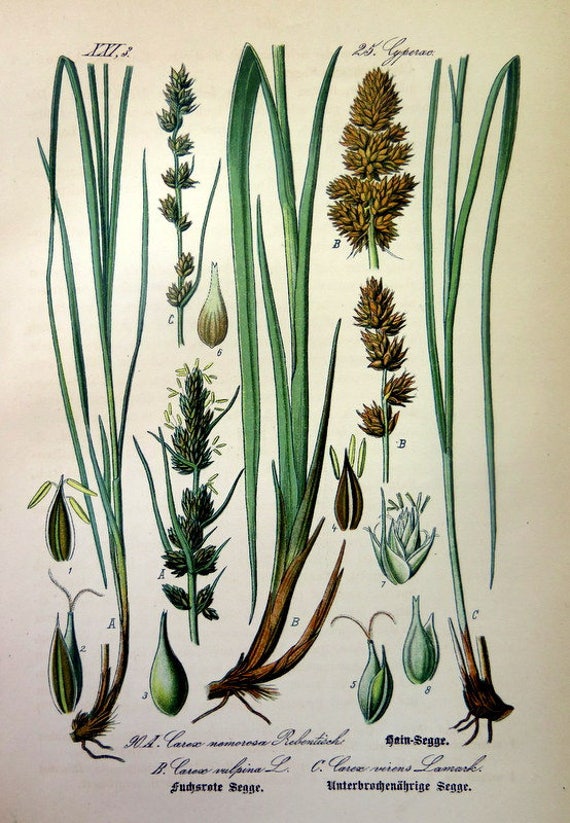This detailed illustration features a tan background adorned with a variety of meticulously drawn plants. From the top of the illustration, a label reads "25, Cyprek" in elegant script, highlighting a green, long grass with visible roots. Additionally, some brown, flowering, weed-like plants are labeled with the letter "B," while "C" denotes a smaller variant of the same plant, characterized by small brown leaves and a green stem. Central to the image is a small object resembling a clove of garlic.

On the lower left corner, there are green, avocado-shaped plants decorated with brown stripes and small leaves sprouting from them, mirrored by similar plants on the right. Each plant within this collection is either numerically or alphabetically labeled for identification (e.g., 1, 2, 3, A, B, C).

The plants are depicted in various stages, from rooting to full sprouting. The colors in the illustration are primarily shades of green and brown, with accents of light brown, light green, and white, adding depth and realism to the botanical details.

Adding a touch of sophistication, the illustration features beautifully handwritten text in a style resembling calligraphy or Old English font, possibly in a foreign language such as German. At the bottom, inscribed in an elegant script, it reads "Sud Srate Sege" (S-E-G-G-E), enhancing the historical and artistic value of the piece.